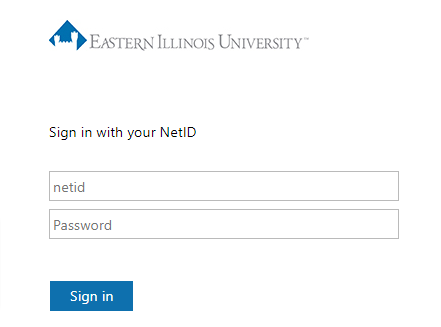In the image, we see a login page for Eastern Illinois University. At the top, the university's name is prominently displayed in gray text alongside a blue diamond containing a white castle-like icon. Below this header, black text instructs users to "Sign in with your Net ID." Further down are two rectangular fields with gray borders; the top field is labeled "Net ID" and the bottom is labeled "Password." Beneath these fields is a blue rectangular button with the words "Sign In" in white text. The entire background of the page is white, providing a clean and simple backdrop that extends from the top to the bottom of the image.